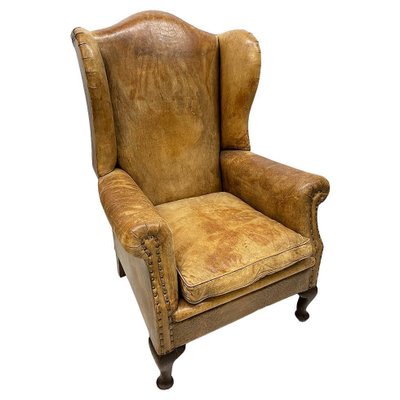The image depicts a well-worn, brown leather wingback armchair against a bright white background. The chair features a high, slightly darker sway back, with rolled armrests adorned with brass grommets or tacks that secure the leather upholstery. The leather exhibits different shades of brown, indicating wear and discoloration, particularly on the removable seat cushion which appears lighter than the rest of the chair. The chair's four wooden legs start wide and taper towards the ground. The design includes subtle indentations on the arms, and a soft padding covers the armrests. There's a noticeable reflection of light at the top of the chair, adding to the unique character of the piece.